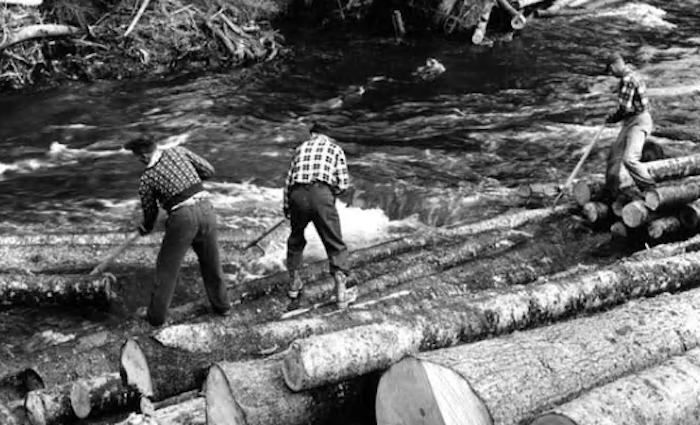In this black and white photo, three men are standing on a pile of long, bark-covered logs on the edge of a fast-moving creek or river, whose foamy white waves indicate its activity. Each man is holding a long pole with a hook at the end, resembling broomsticks or claw-like sticks, used to pull the logs from the water. The two men on the left are actively engaging with different logs in the water, suggesting a coordinated effort to manage the floating lumber. The man on the right, however, appears without a log to handle at the moment. They're all wearing checkered sweaters, although the exact colors cannot be discerned due to the monochrome palette. In the background, the far bank of the creek is visible, adorned with shrubbery and potentially a tree on the upper right-hand side. This serene yet industrious scene captures the essence of early log transportation and the challenging work environment of loggers.